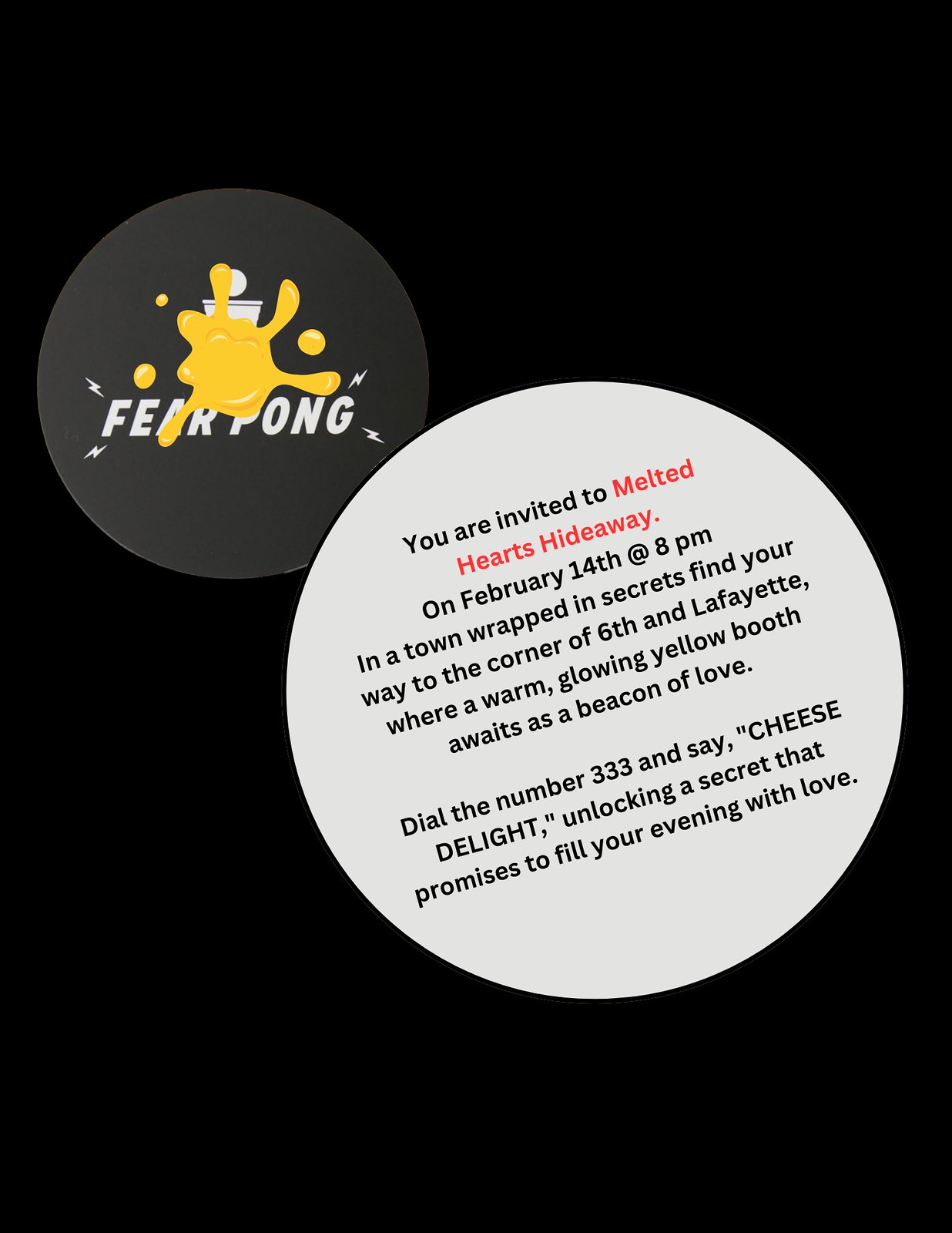The image showcases a striking advertisement set against a solid black background. Dominating the right side of the image is a large white circle containing red and black text, extending an invitation to "Melted Hearts Hideaway" on February 14th at 8 p.m. The detailed invitation reads, "You are invited to Melted Hearts Hideaway on February 14th at 8 p.m. in a town wrapped in secrets. Find your way to the corner of 6th and Lafayette where a warm glowing yellow booth awaits as a beacon of love. Dial the number 333 and say Cheese Delight, unlocking a secret that promises to fill your evening with love." To the upper left is a smaller black circle with white text that says "Fear Pong," partially obscured by a vibrant yellow splatter. Atop this circle, a cup with a ball resting on it is depicted, surrounded by small yellow lightning bolts in each of the corners of the word "Fear Pong," and a yellow paint splash above. The contrasting colors and playful elements suggest a Valentine’s Day event filled with intrigue and excitement.